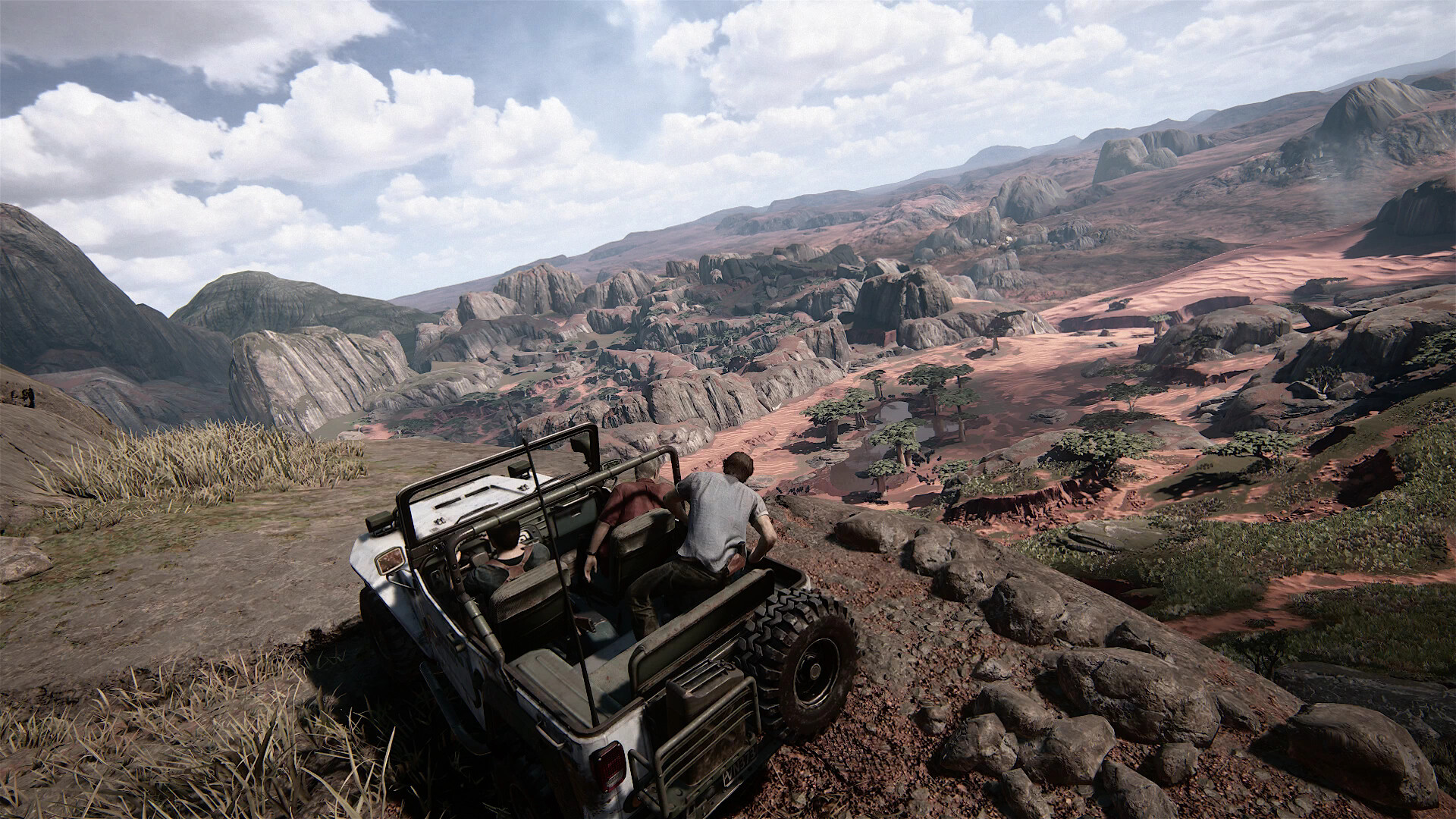In this striking aerial photograph, a topless Jeep is perched majestically atop a mountain, offering an awe-inspiring view into a sprawling canyon below. Captured from a high angle behind the vehicle, the image reveals three men seated inside the Jeep. The man in the back seat sports a gray short-sleeve shirt and black hair, while the passenger on the right wears a brown short-sleeve t-shirt and has grayish hair. The driver, with black hair and clad in a greenish-gray shirt, appears focused as all three men gaze intently over the edge, seemingly captivated by the breathtaking scenery that stretches out before them.